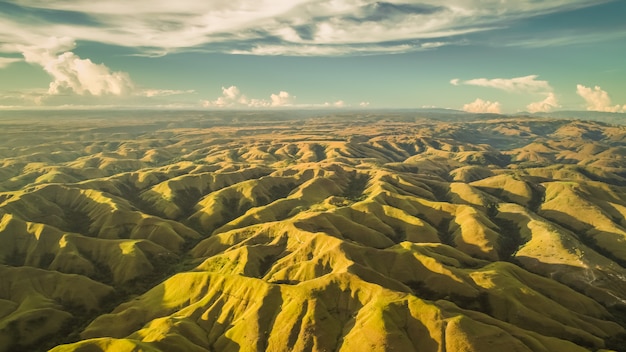The image depicts an aerial view of an expansive desert mountain range, stretching endlessly into the distance. The terrain is composed of weather-beaten, gold-hued mountains, their peaks and valleys interlocking and creating deep shadows that accentuate the rugged topography. The mountains, possibly foothills due to their modest size, are corroded and carved by erosion, presenting a landscape rich in grooves and contours. Above, the midday sky is a clear, vibrant blue, interspersed with numerous white clouds, particularly concentrated along the horizon and the upper portions of the frame. The golden light of the sun casts striking shadows down the sides of the mountains, enhancing the scene's dramatic and almost ethereal beauty. The vast sprawl of mountaintops dominates the composition, projecting an endless, weathered expanse beneath the slightly overcast sky.